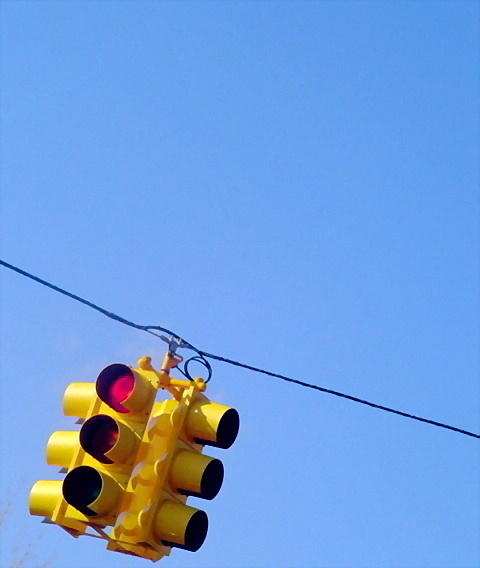The image captures a standard traffic light against a bright, cloudless midday blue sky. Taken from below, the photograph reveals a red-yellow-green signal with yellow housing, hanging at an angle from a twisted wire running from the center left to the lower right of the frame. Despite the traffic light being centered in the image, its alignment is noticeably skewed, possibly due to high wind. The visible red light faces the left, while the remaining traffic lights are oriented towards different directions. In the lower left corner, there are bare branches of a tree. The clear, vibrant blue of the sky and the angular suspension of the traffic light add dynamic elements to the composition.